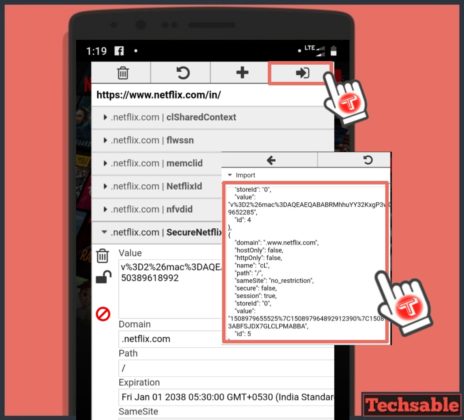This image features a black border with a pinkish-salmon colored background. Central to the composition is a cell phone with its screen turned on. The status bar at the top of the screen indicates a notification count of 119 next to the Facebook icon on the left, and signals LTE connectivity alongside a battery icon on the right.

On the screen, a series of icons appear: a trash can, an arrow, a circle with a plus sign, and an arrow pointing to the right inside a red box. The image of a hand, specifically an index finger pointing towards the red-bordered box, is prominently featured. On the hand's index finger is a red circle containing the letter 'T.'

Beneath this, the screen displays a URL for Netflix in India, formatted as "netflix.com, CL, shared content." It includes additional Netflix addresses such as "LWSSN" after "netflix.com." Further down, a variety of symbols and text are visible, including another trash can, the word "value," an open padlock, and a string of numbers and letters. There is also a red circle with a line through it next to the text "domain.netflix.com," with an expiration date listed as Friday, January 1, 2038, noting the time in India Standard Time. 

A red-bordered box filled with domain information, including terms like "post only" and various paths, numbers, letters, and symbols, is present. Finally, in the bottom corners of the screen, the word "techsable" appears, completing the detailed and technical display depicted on the cell phone screen.